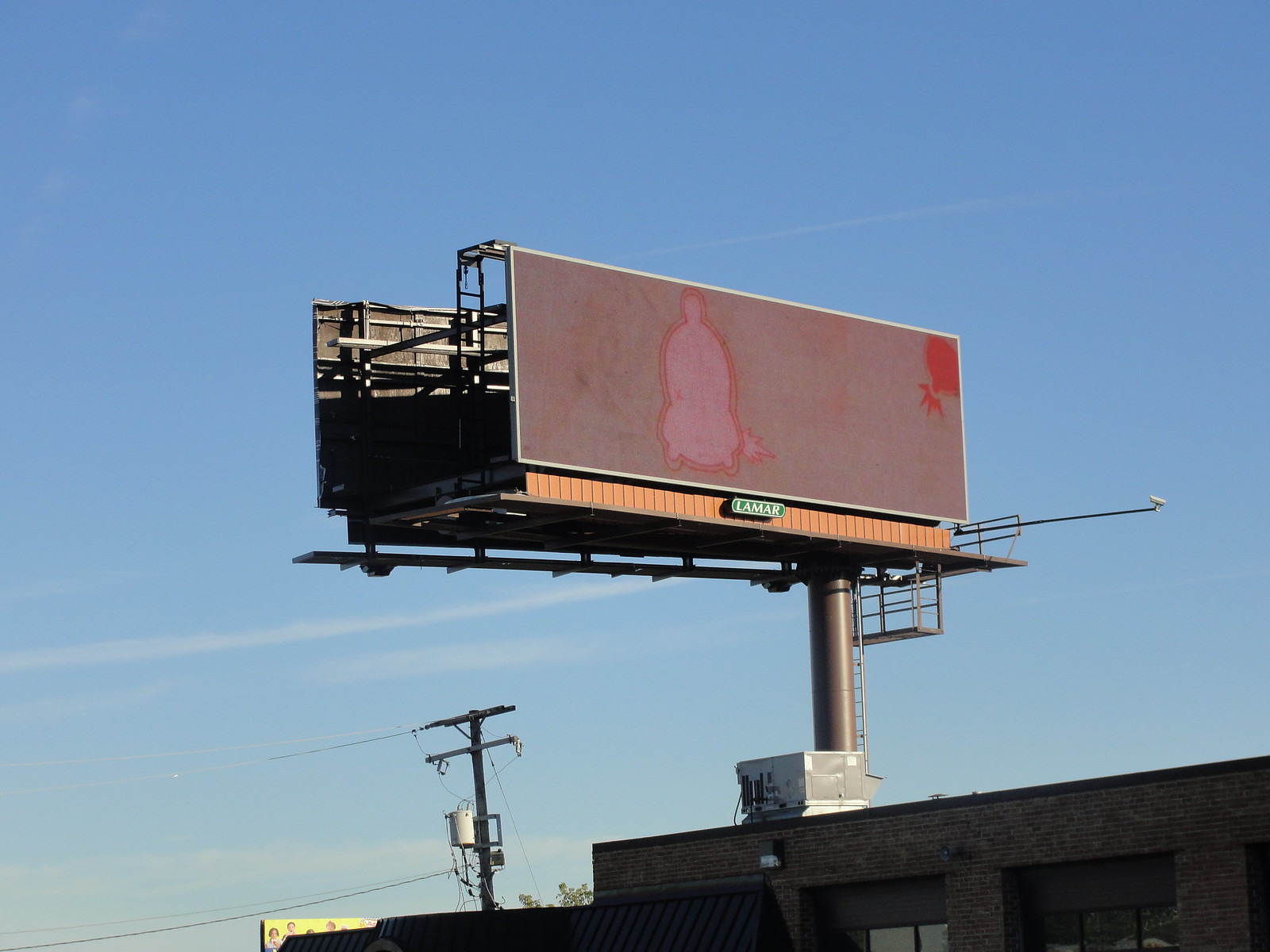In this photograph, a partially obscured billboard emerges, creating the illusion that it is sprouting from the top of a building. Against a backdrop of a clear blue sky, the left side of the scene features several electric posts. The billboard is branded with "Lamar" at its base and exhibits a muted mauve background devoid of text. Intriguingly, an orange circle with a partial ray in the upper right-hand corner suggests the presence of the sun. Towards the middle-left of the billboard, there is a pink silhouette that bears a resemblance to a human figure, characterized by a small head and a broader body below. The figure appears to be seated cross-legged, conjuring images of someone dressed in robes. Further adding to the mystique, a small, spiky protrusion extends from the bottom side of the silhouette. This ambiguous shape invites multiple interpretations, sparking curiosity and imagination regarding its true nature.